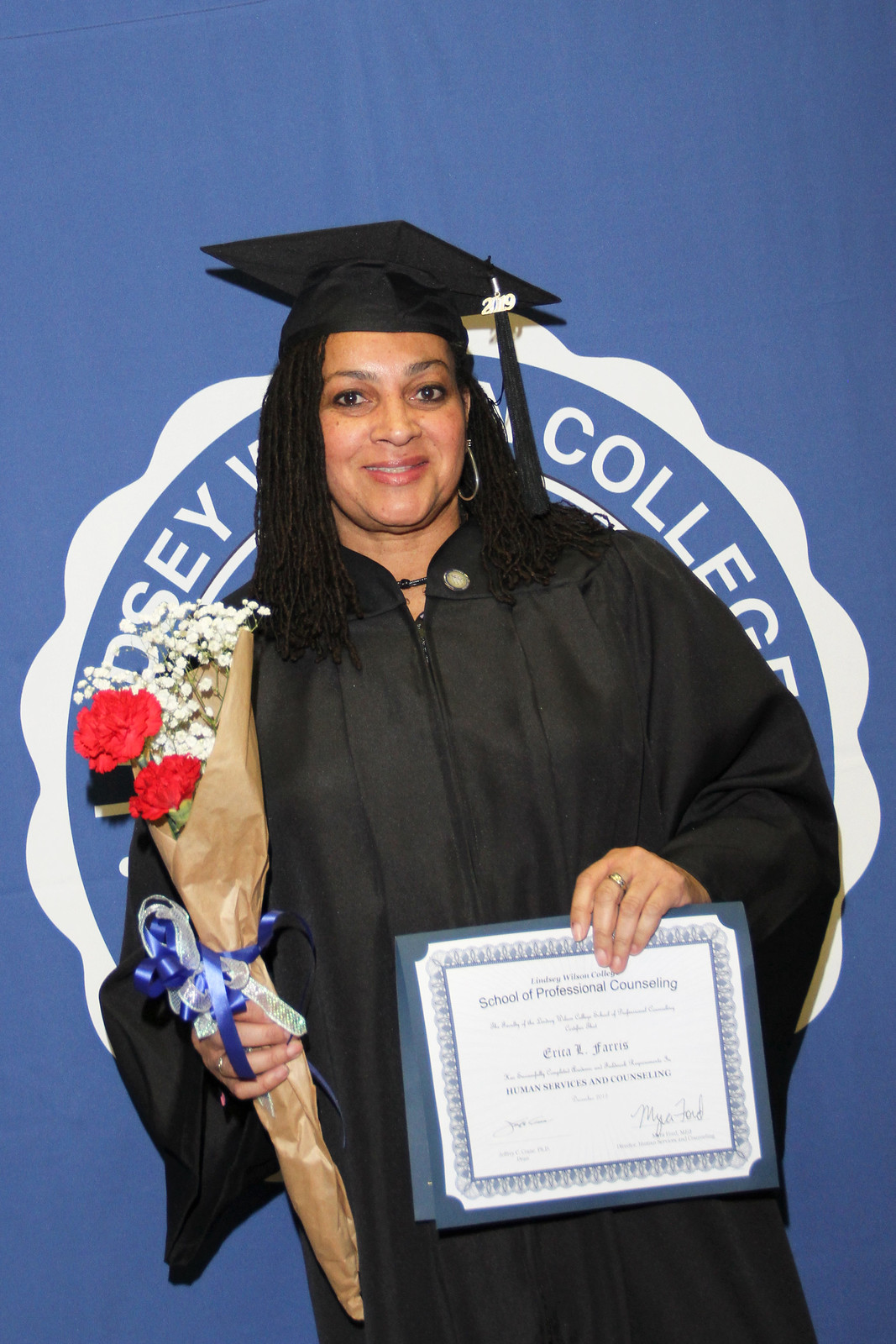This photograph captures a smiling woman, likely in her 30s or 40s, celebrating her graduation. She is adorned in a black graduation cap with a black tassel that says "2019", and a traditional black gown. Her dark black, thin braided hair frames her joyful expression. In her left hand, she proudly holds a blue and white diploma from the School of Professional Counseling, Human Services and Counseling, bearing the name Erica R. Farris. In her right hand, she carries a beautifully arranged bouquet of red roses and baby's breath, wrapped in light brown paper and tied with a blue and white ribbon. She wears a ring on her left ring finger. Behind her is a blue backdrop featuring a circular insignia partially blocked by her head, but identifiable as belonging to her college. This backdrop and her academic regalia create a fitting and celebratory scene for her achievement.